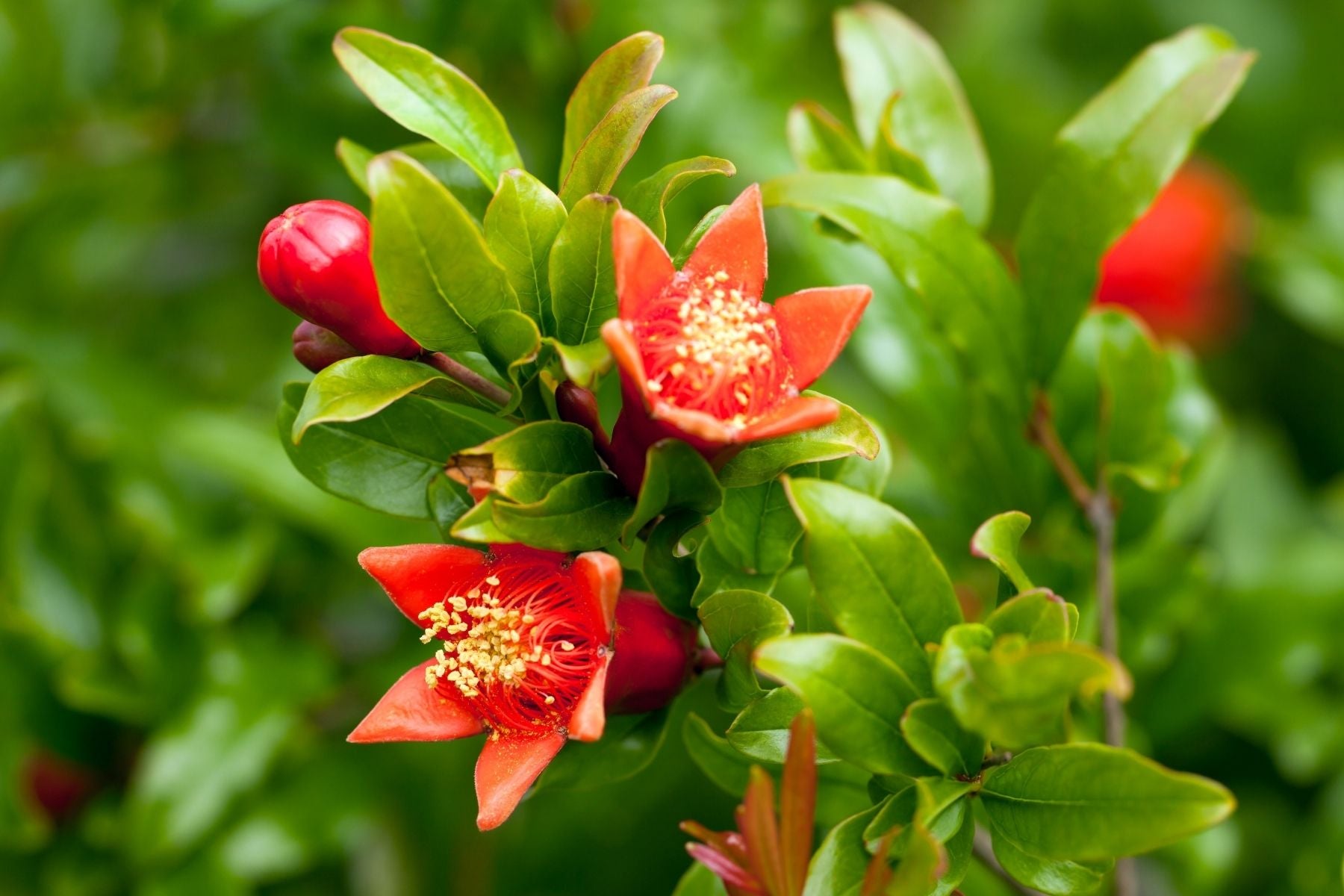The image displays a detailed close-up of two fully grown white flowers, each adorned with six red petals and numerous red filaments topped with yellow tips. Positioned centrally and towards the lower left bottom of the frame, these blossoms are framed by an abundance of thick, shiny green leaves that fill the background. Near the top left, there are several bulbs yet to open, hinting at more blooms to come. The intricate design of the red petals, with their jagged, interlocking edges, suggests a unique mechanism where the petals close together. The rich texture and vivid colors of the flowers, coupled with the lush green foliage, create a strikingly detailed and vibrant botanical scene.